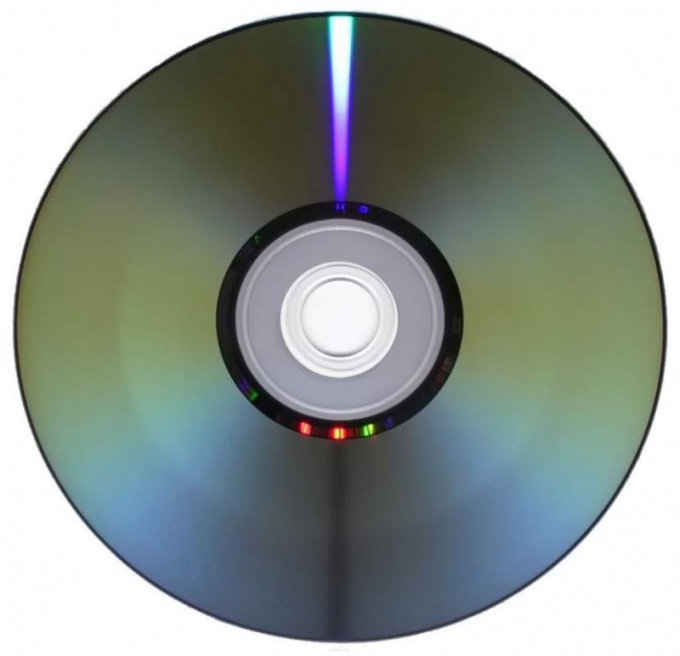This image is a detailed, close-up view of the bottom side of a compact disc, set against a stark white background. The disc features a clear plastic center with a small, central hole, typical for mounting onto a Discman or a computer tray. The inner ring surrounding the hole has a black coloring, creating a distinct border between the clear center and the reflective data layer. This data side of the CD showcases its characteristic metallic sheen, with a gradient streak of light stretching from bright purple at the bottom to bright blue at the top. Additionally, reflections of green and red light are visible in some of the more reflective areas, enhancing the glossy and polished appearance of the disc.